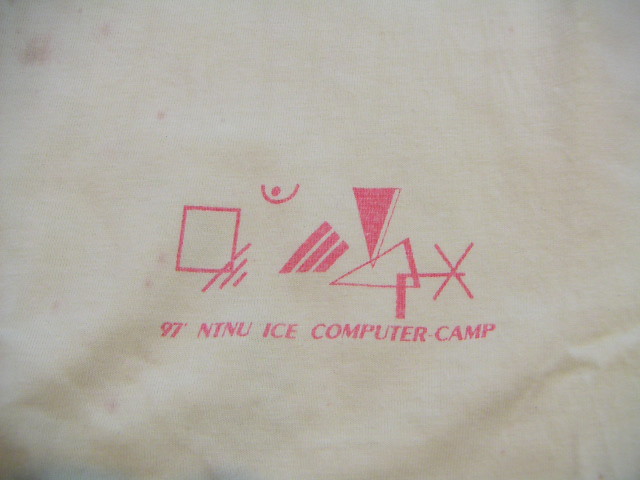The image is minimalistic, featuring a slightly crumpled white piece of paper with pink text prominently displayed. The printed text reads "97 NINU NTNU ICE Computer Camp." Positioned above the text, there is a square containing three thin, diagonal lines, with the longest line extending through and beyond the square. To the right of the square are three thick diagonal lines, each touching the other and forming a cluster. The cluster comprises a pink triangle with a white border, a white triangle with a pink border, and another white triangle, which are placed in close proximity to one another. Adjacent to these elements is a bold 'X' symbol, completing the design. The overall composition is straightforward, yet it combines various geometric shapes and typographical elements in a visually interesting manner.